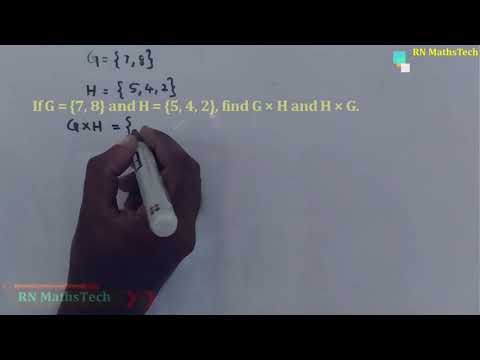The image is a detailed screenshot from a video showcasing a mathematical lecture or tutorial. Central to the image is a whiteboard filled with numerical and algebraic formulas, written in black marker. A hand, likely of an instructor, is seen writing on the whiteboard, holding the black marker between its fingers. Superimposed on the whiteboard, in yellow text, is the equation: "If G = (7, 8) and H = (5, 4, 2), find G × H and H × G." Additionally, the top right corner features the text "RN Maths Tech" in yellow, alongside a light blue square with a smaller white square beneath it. The bottom left corner also displays the watermark text "RN Maths Tech" in blue. The entire image is bordered by a long black bar running across both the top and bottom.